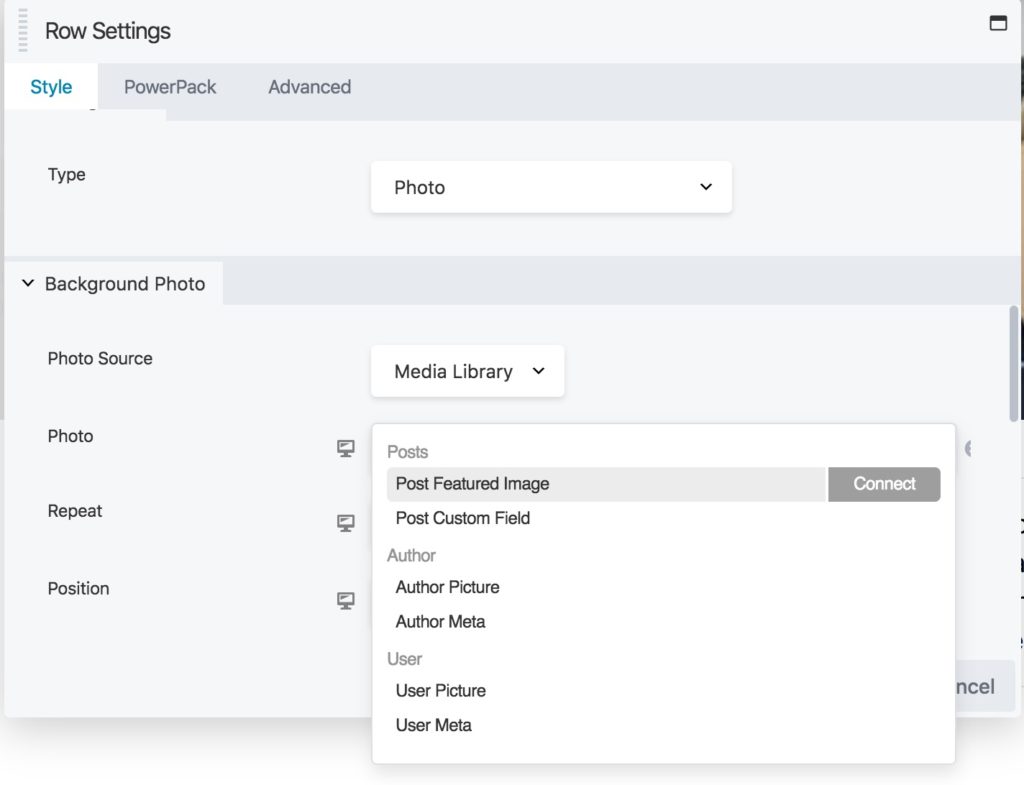In the photographic image, an application interface is depicted prominently at the top of the page. A light gray banner features black text that reads "Row Settings." To the right of this text, there is an icon representing a folder. Below this banner, blue text indicates that the "Style" tab is selected and currently open. Adjacent to this on the gray tab are other selectable options titled "PowerPack" and "Advanced."

Within the "Style" tab, various settings are displayed. The "Type" setting, indicated as selected, includes a drop-down menu with an arrow pointing downward, showing that "Photo" has been chosen. Further down, another drop-down under "Background Photo" shows that the "Photo Source" is set to "Media Library."

Additional settings include options for "Photo Repeat" and "Position," each accompanied by an icon resembling a monitor. Beneath these, a series of post-related settings are listed. "Post Featured Image" is visibly selected, with the option to connect via a gray button. Other post-related options include "Post Custom Field," "Author" (with sub-options "Author Picture" and "Author Meta"), and "User" (with sub-options "User Picture" and "User Meta").